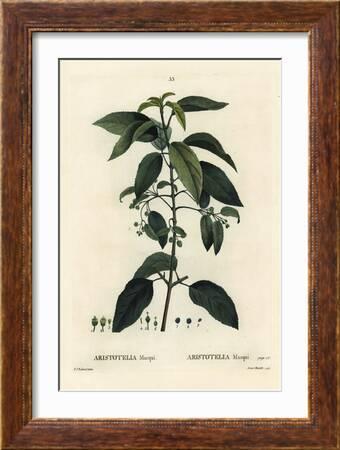The image showcases a framed botanical illustration, encased in a dark stained, rectangular wooden frame. The frame is complemented by a pristine white matting that borders the artwork. The illustration itself is rendered on a cream or vellum-colored background, suggesting an antique or older piece. At the center of the illustration, a long leafy stalk, possibly from a tree or shrub, extends upward from the bottom and curves gracefully to the left. The stalk is adorned with numerous ovate green leaves and features small panicles of white flowers. Some fallen leaves rest near the base of the stem. There is also some faint, indecipherable writing at the bottom of the illustration, which typically indicates the type of plant depicted, reminiscent of botanical illustrations found in herbariums.